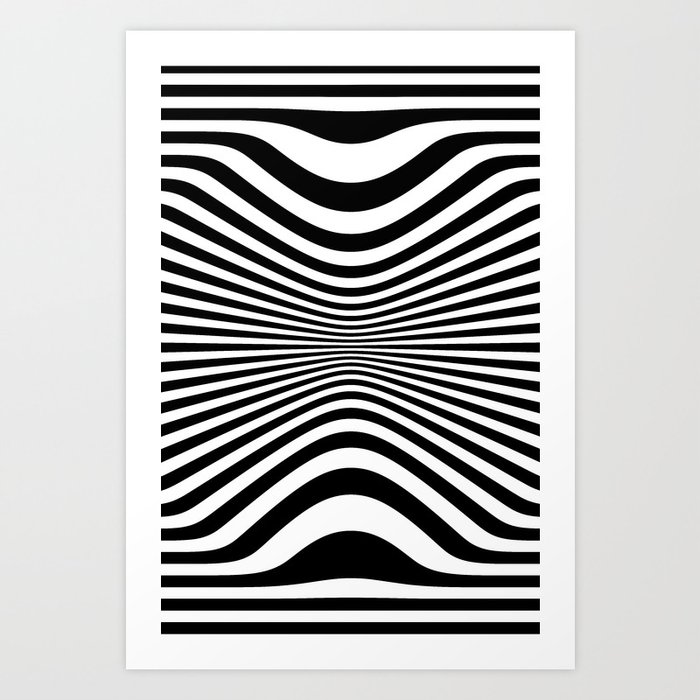The image appears to be either computer-generated or a photograph of an art piece, possibly on display in a museum due to its immaculate presentation on a white wall. The artwork itself is a striking black and white poster, approximately five feet tall and four feet wide, that exudes a strong optical illusion. The piece features an arrangement of horizontal black stripes of varying sizes and shapes which create a mesmerizing 1960s psychedelic effect. At the top and bottom of the image, the lines begin straight, but as they progress towards the center, they develop curves and undulations, some swelling and shrinking in size. This intricate interplay of lines creates a visual effect that makes the image appear to pulsate and move, drawing the viewer's eye inward towards the center where the lines become more tightly compacted, further enhancing the illusion of depth and movement. The artwork is reminiscent of a zebra's stripes due to its black and white palette, and the overall visual complexity evokes the sensation of looking at an animated and dynamic piece of modern art.